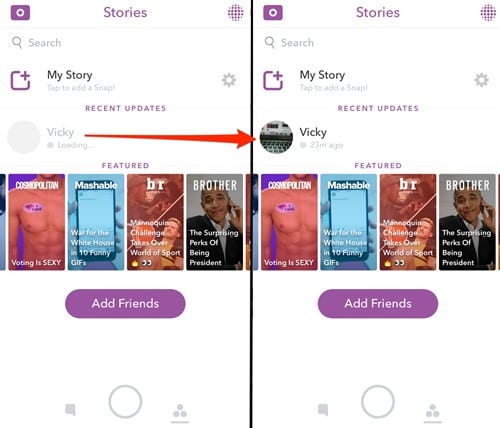The image depicts two screenshots of a smartphone interface, which appear to be from the Snapchat app. 

On the left screenshot, the top of the screen says "Stories," alongside a purple square icon with a circle inside it. Below, there’s a search bar displaying "My Stories" with a prompt to "Tap to add a snap," followed by a settings icon on the right. Under the "Recent Updates" section, it mentions "Vicki's Vicki loading" and a red arrow pointing towards the right screenshot.

The right screenshot shows a similar layout, but under the "Recent Updates" section, it says "Vicki 21 minutes ago," accompanied by her profile icon in a circular shape, which is absent in the left screenshot. The text and background color for this section is gray, contrasting with the black background in the left screenshot.

Below both screenshots, there's a section of four vertically arranged rectangular icons displaying various media stories such as "Cosmopolitan: Voting is Sexy," and other stories by "Mashable," "BI," and another by "Mashable." At the bottom, there is a purple button labeled "Add Friends," next to an icon resembling a speech bubble accompanied by three circles, representing additional options or features.